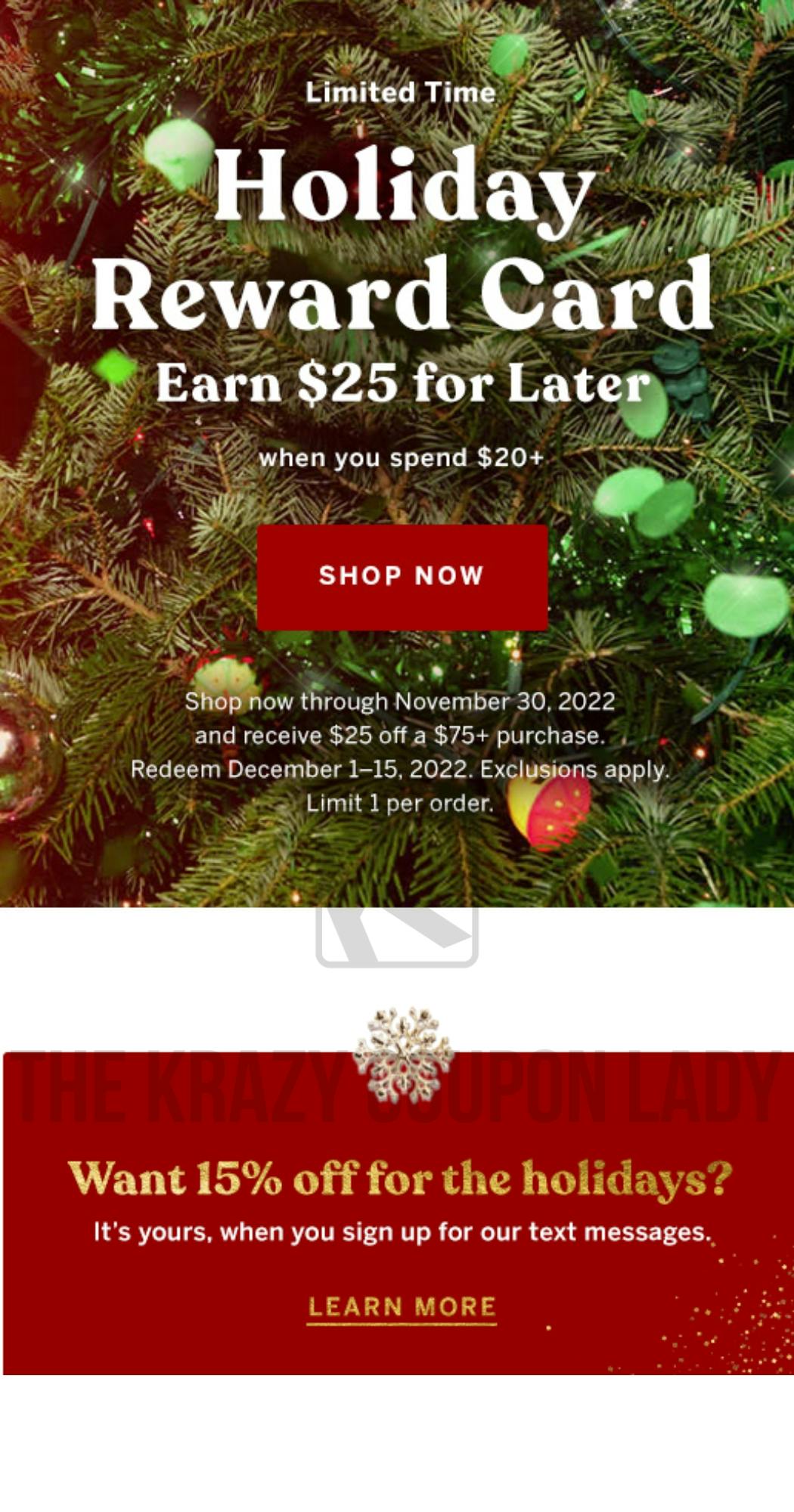Screenshot of an advertisement: At the top, there is a photograph of a close-up Christmas tree featuring green evergreen pine boughs adorned with digitally added, unattractive green lights. The text overlay in white font reads, "Limited Time Holiday Reward Card." Below this, it states, "Earn $25 for later when you spend $20+."

Underneath this message, a red rectangle with white font prompts viewers to "Shop Now." Further down, another line reads, "Shop now through November 30, 2022, and receive $25 off a $75 purchase, redeem December 1-15, 2022. Exclusions apply. Limit one per order."

A light bar separates this section from another red rectangle below. This rectangle displays the brand name "The Crazy Coupon Lady" in translucent gray. In yellow font, a message asks, "Want 15% off for the holidays?" Beneath this, white font informs, "It's yours when you sign up for our text messages." Finally, another prompt in yellow font states, "Learn More."